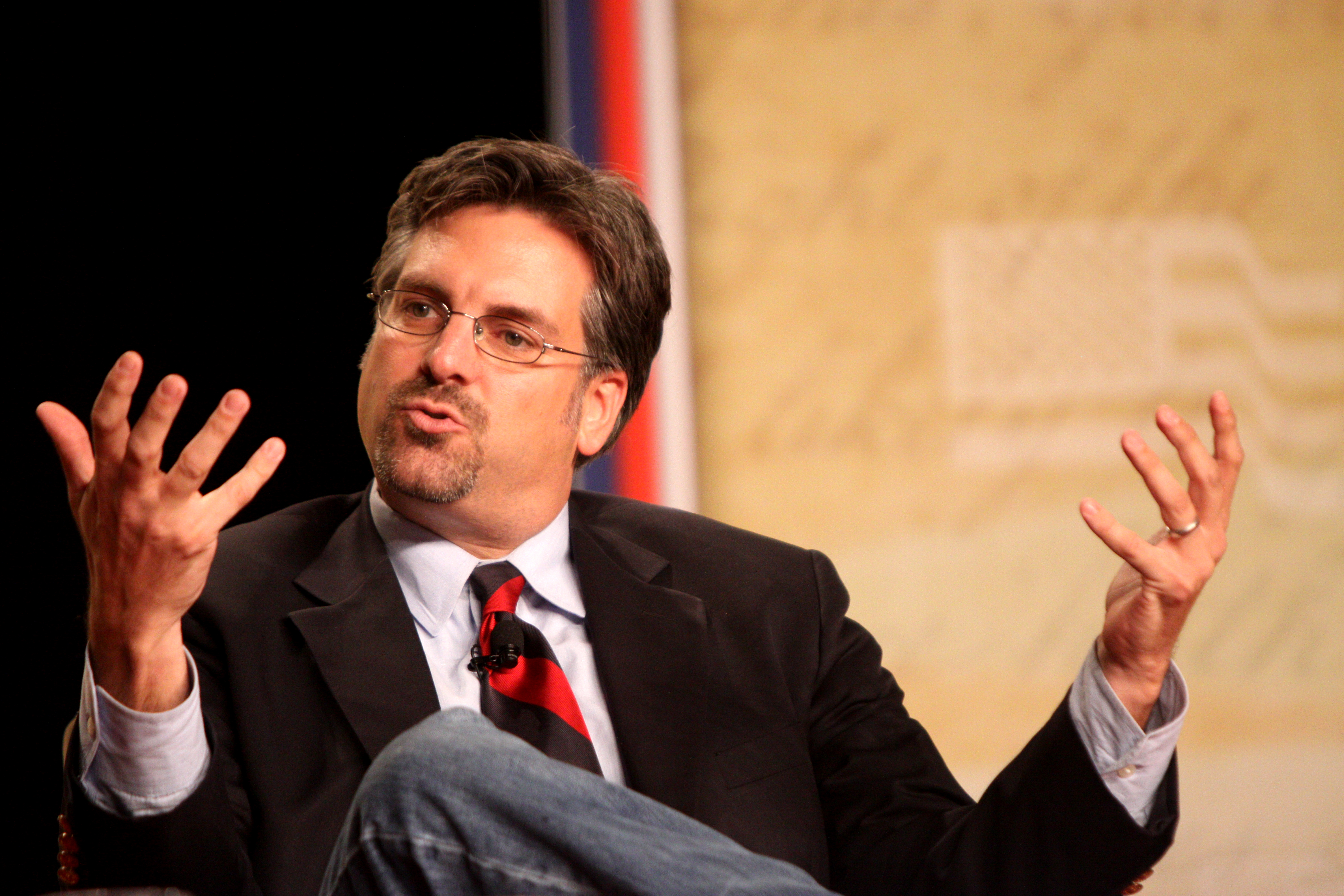In this detailed photograph, we see a slightly heavyset Caucasian man, likely aged between 40 and 45, seated and engaged in a conversation or debate, with an expressive demeanor evident from his raised and gesturing hands. His hands, palms up, suggest he is in the midst of explaining or imploring something to an off-camera audience positioned to the left of the frame. The man, who has shorter brown hair with some salt and pepper, is wearing wire-rimmed glasses and sports a light goatee and mustache.

He is dressed in a black blazer over a light blue, long-sleeve collared shirt, with a red and black striped tie. Despite the formal attire on his upper half, he is notably wearing blue jeans, visible due to his ankle being crossed over his opposite knee. Additionally, he has a microphone clipped to his tie and a wedding band on his fourth finger of his left hand. 

The backdrop of the image features the superimposed imagery of the American flag and what appears to be the handwritten version of the Declaration of Independence, commonly used as a backdrop in political settings. The background remains blurred but recognizable enough to suggest a politically charged or formal event setting. The photo captures a candid moment, emphasizing the intensity and casual formality of the man’s participation in the event.